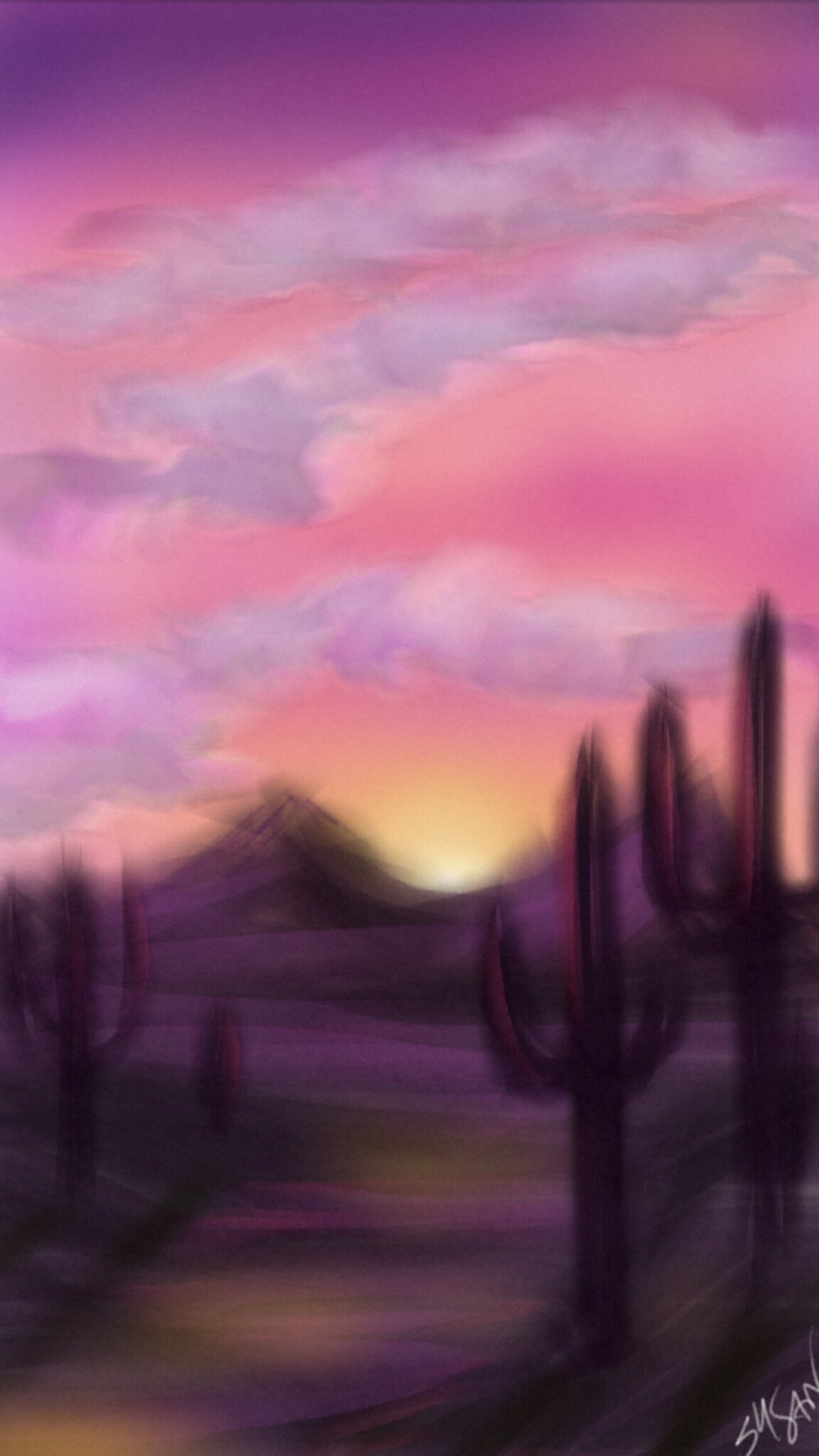The image depicts a vertically rectangular, blurred artwork, possibly an oil painting with watercolor-like smudging effects. The scene portrays a dramatic desert sunset. At the top of the frame, the sky transitions from dark purple to pink, and finally to a glowing orange near the horizon, accentuated by three bands of whitish-pink clouds stretching horizontally. The sun sets between two large, dark purple mountains adorned with black and dark green accents.

The foreground features a path with a blend of light brown and purple hues, illuminated diagonally by the remaining sunlight. On the right side, two tall, black cacti with red-purple highlights stand prominently. Additional cacti, similarly colored, appear on the left, including one large and one small round cactus. The entire image has a purple tint, heightening the sense of twilight.

In the bottom right corner, the artist's name "Sai San" is inscribed in white, albeit faintly legible.